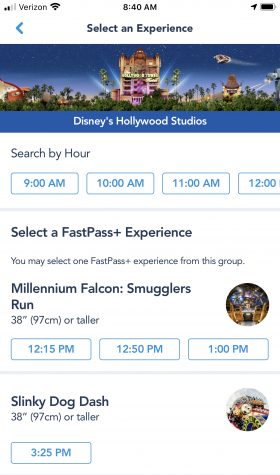The screenshot displays various information from a smartphone screen related to booking FastPass experiences at Disney's Hollywood Studios. 

In the upper right-hand corner, the battery icon shows nearly full battery life. The current time is indicated in the center of the screen, reading 8:40 AM, while the upper left-hand corner shows the mobile carrier as "Verizon."

The main content of the screenshot includes a section for selecting an experience at "Disney's Hollywood Studios." Above this visual, there is a heading that says "Select an Experience," and below it is an option labeled "Search by hour," followed by boxes representing different hours: 9 AM, 10 AM, 11 AM, and 12 PM, though the list is cut off at this point.

The area beneath these search options contains a detailed section for selecting a FastPass+ experience. It instructs users that they may choose one FastPass+ experience from the provided group. 

First on the list is "Millennium Falcon: Smugglers Run," which has a height requirement of 38 inches (97 centimeters) or taller. There are three available time slots for this experience: 12:15 PM, 12:50 PM, and 1:00 PM. 

Following this, the next available experience is "Slinky Dog Dash," also with a height requirement of 38 inches (97 centimeters) or taller. The only available time slot for this attraction is 3:25 PM.

The background of the screenshot is white, providing a clear and clean layout for the various interactive elements and text.